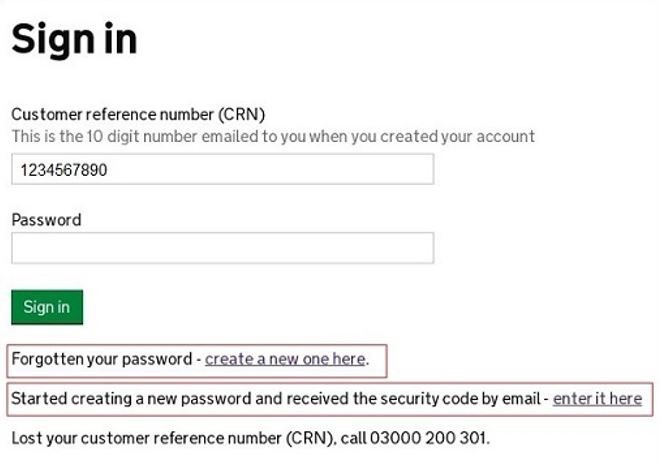The image displays a sign-in screen with detailed instructions and fields for user entry.

At the top left, the screen is titled "Sign In" in bold black lettering. Below this heading, in smaller black lettering, it reads "Customer Reference Number (CRN)". Underneath this, there is a line of light gray text explaining, "This is the 10-digit number emailed to you when you created your account." 

Following the description, the first input field appears as a light gray bordered elongated rectangle, meant for users to enter their customer reference number; an example "1234567890" is shown in black lettering within the field. Beneath this is another label "Password" in black lettering, accompanied by another editable field for password input.

Below these input fields, there is a smaller button in a dark mossy green color with "Sign In" written in white lettering. Beneath this button is a red-bordered rectangle containing black text that reads, "Forgotten your password - create a new one here." The phrase "create a new one" is displayed in dark purple, indicating a previously visited link.

Further down, another longer red-bordered rectangle offers instructions for users who have started creating a new password and received a security code by email. The text says, "Started creating a new password and received the security code by email - enter it here," with "enter it here" also in dark purple, indicating it has been clicked before.

At the bottom of the screen, there is guidance for those who have lost their Customer Reference Number (CRN), stating, "Lost your Customer Reference Number (CRN)? Call 0300 200 301." The phone number is clearly spaced for easy reading.

This layout helps users navigate the sign-in process efficiently, offering clear options for retrieving lost information and continuing with account access.